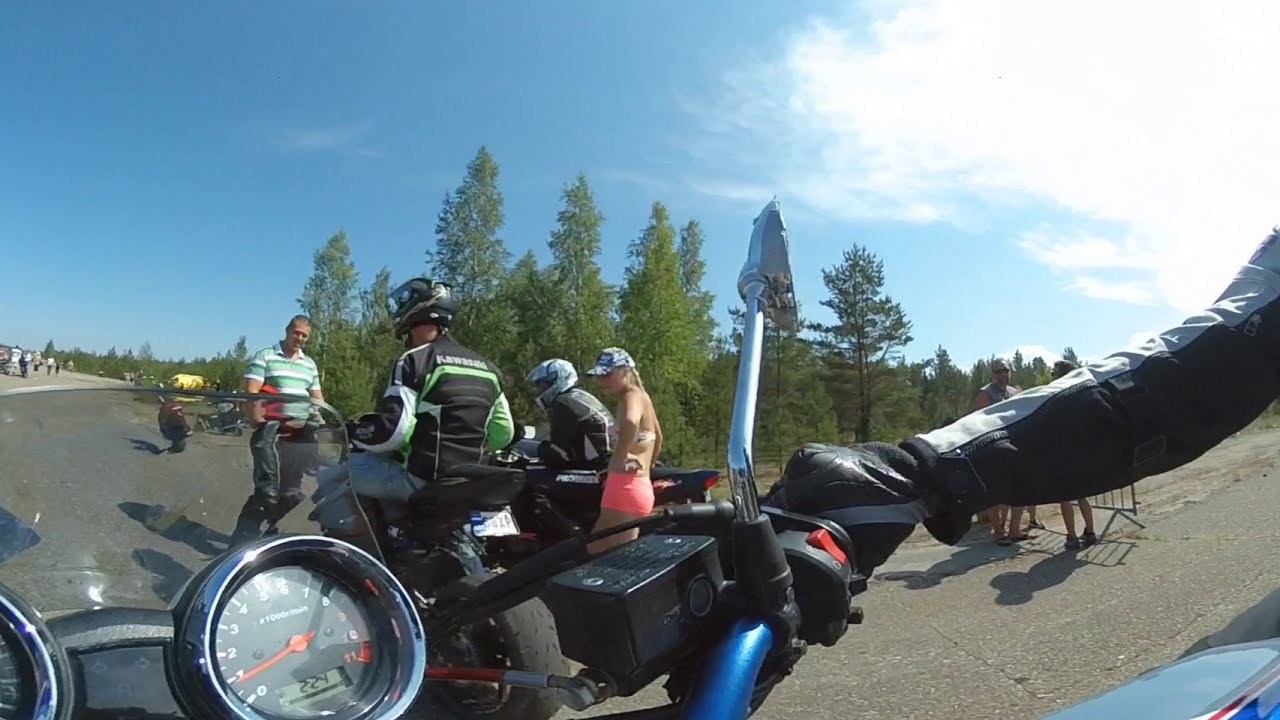The image is a panoramic, slightly wide-angle shot from the perspective of a motorcyclist. In the foreground, we see the cockpit of the motorcycle, featuring the RPM gauge, windshield, right handlebar, and mirror, along with the right arm of a rider wearing a black and white jacket and shiny black gloves. The scene is outdoors, along a road or parking lot bordered by trees and a small fence. Several people are gathered around the area—two or three motorcyclists, including a person in a black and white helmet, and a woman in a bikini top, coral-colored shorts, and a black and white baseball hat. A man in a green and white striped shirt and jeans appears to be approaching the group. The backdrop reveals a partly cloudy, almost clear, blue sky, indicating a likely non-winter season with the trees fully green.